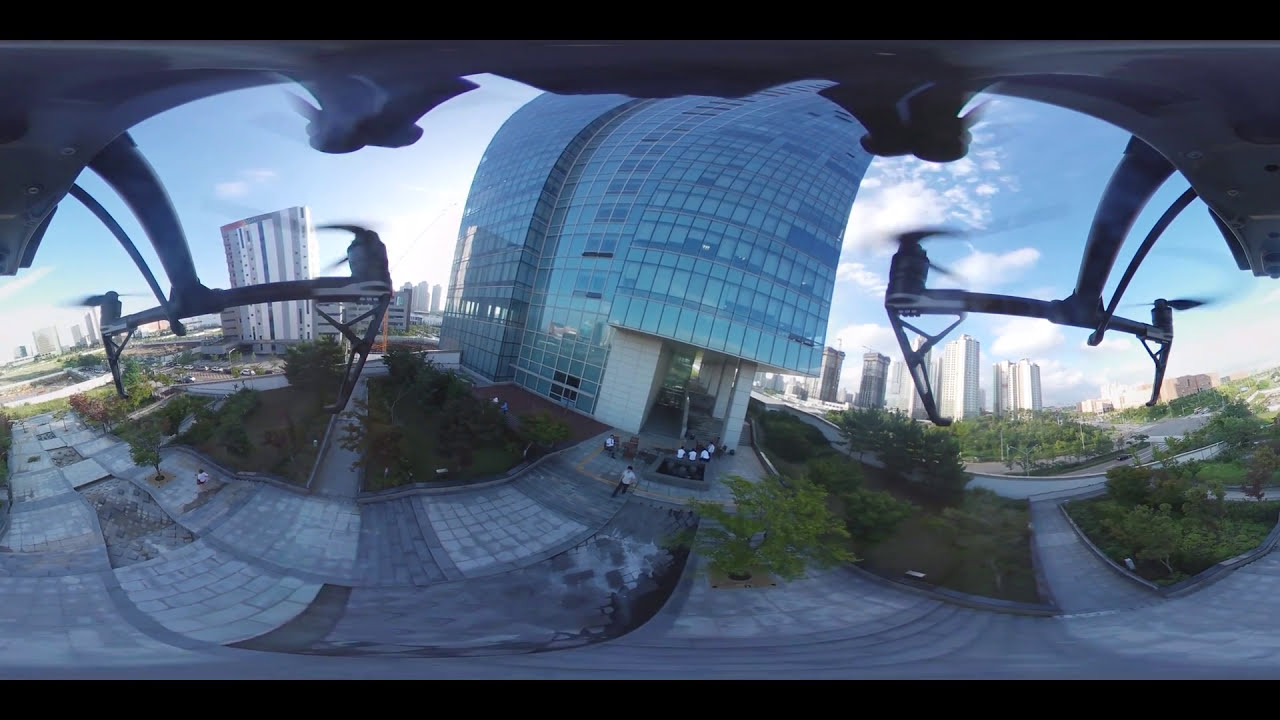The image captures a vibrant urban scene from the perspective of a small DJMAF drone, flying around one to two stories above ground level next to a glass-clad skyscraper. The drone's rotors and struts are visible in the slightly distorted, possibly 360 panoramic shot, with thin black framing lines at the top and bottom. The bending lines of the image suggest a wide-angle lens effect. Surrounding the main skyscraper is an array of well-manicured, rectangular gardens with grass and trees, contrasting with the concrete tiles below. In the foreground, a few people can be seen walking or sitting, hinting at the photo being taken near a busy commercial or office area. The background showcases a dense cityscape with numerous tall skyscrapers under a sunny, partly cloudy sky. The drone itself has a bluish tint, further adding to the intricate details captured in this dynamic aerial shot.